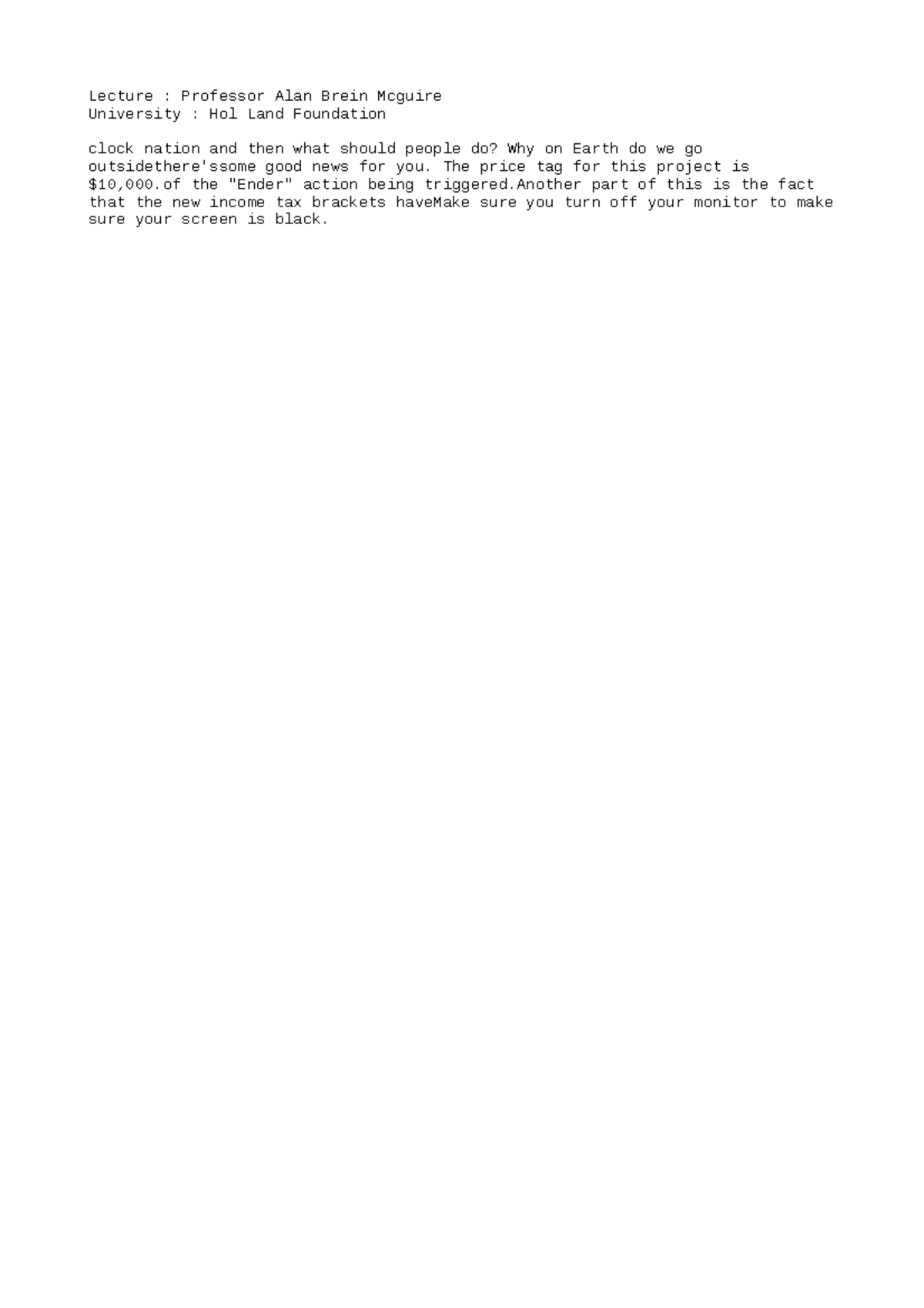This image features plain black text set against a white background. The context of the project references an expense of $10,000 triggered by an ENDA action. Additionally, it notes the recent updates in income tax brackets. To ensure the display integrity, it mentions turning off the monitor to confirm the screen is not illuminated.